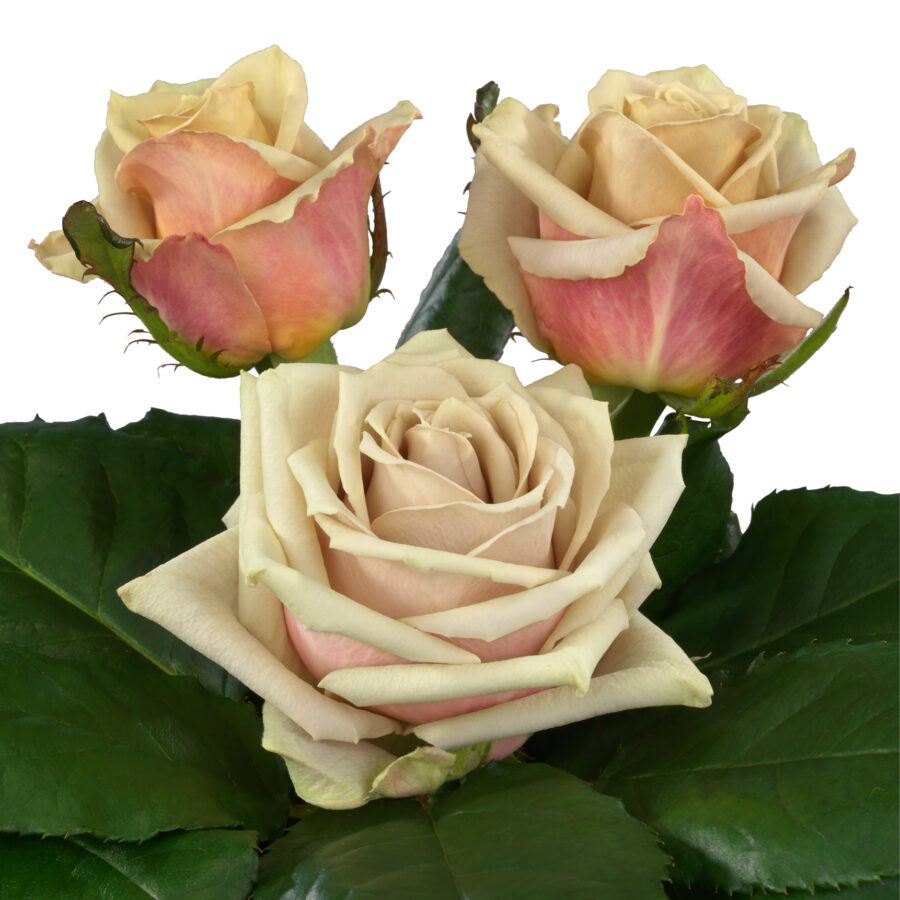The photograph captures three exquisite roses on a bush, delicately blending shades of cream and pink. The largest rose, prominently placed at the front, is more open compared to the two smaller, less open roses situated behind it. Each petal exhibits a graceful transition from cream or white on top to a soft pink on the underside, adding a subtle yet elegant contrast. Surrounding the roses is a lush frame of bright green foliage, with larger leaves at the base providing a vivid backdrop. The image is artistically set against a completely white background, highlighting the roses and their greenery with striking clarity and making the floral arrangement appear almost ethereal and meticulously curated.